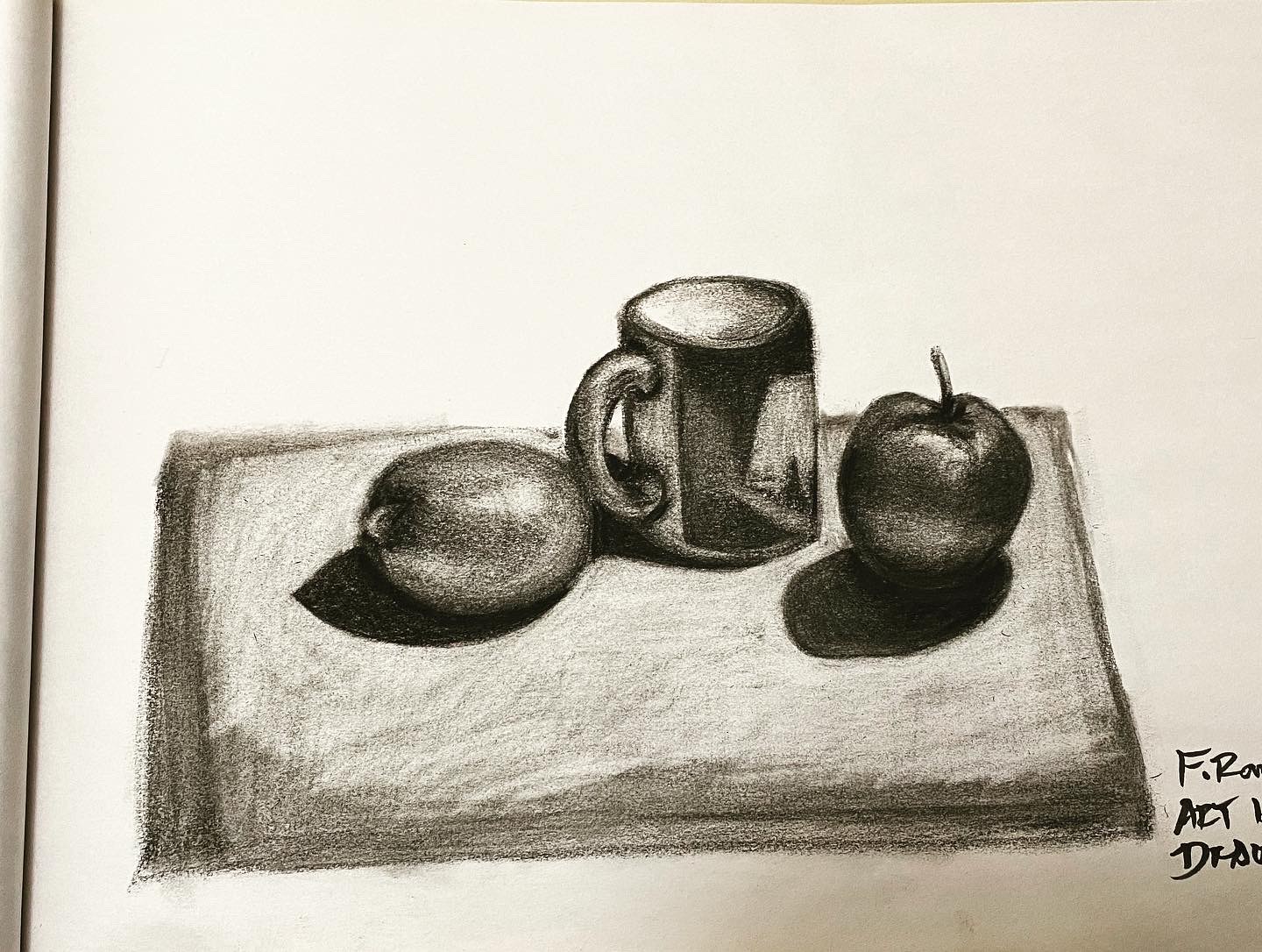This detailed black-and-white sketch, likely executed in pencil or charcoal, illustrates a still life scene featuring a table with two fruits and a mug. Positioned on the left is an oval-shaped citrus fruit, possibly a lemon, its identity suggested by its form. In the center, a sturdy mug stands, and to its right, a distinctive apple can be identified by its familiar shape and stem. The lack of color nuances emphasizes the interplay of light and shadow, casting prominent shadows from the three objects, which add depth and dimension to the composition. On the right edge of the drawing, partially obscured and difficult to decipher, are some textual elements. These appear to read "F.R.O. Act 1" and include another fragmentary inscription beginning with "D.R.," though the cut-off nature of the text makes it hard to fully interpret. The presence of this text suggests additional context or titling pertinent to the artwork's narrative.